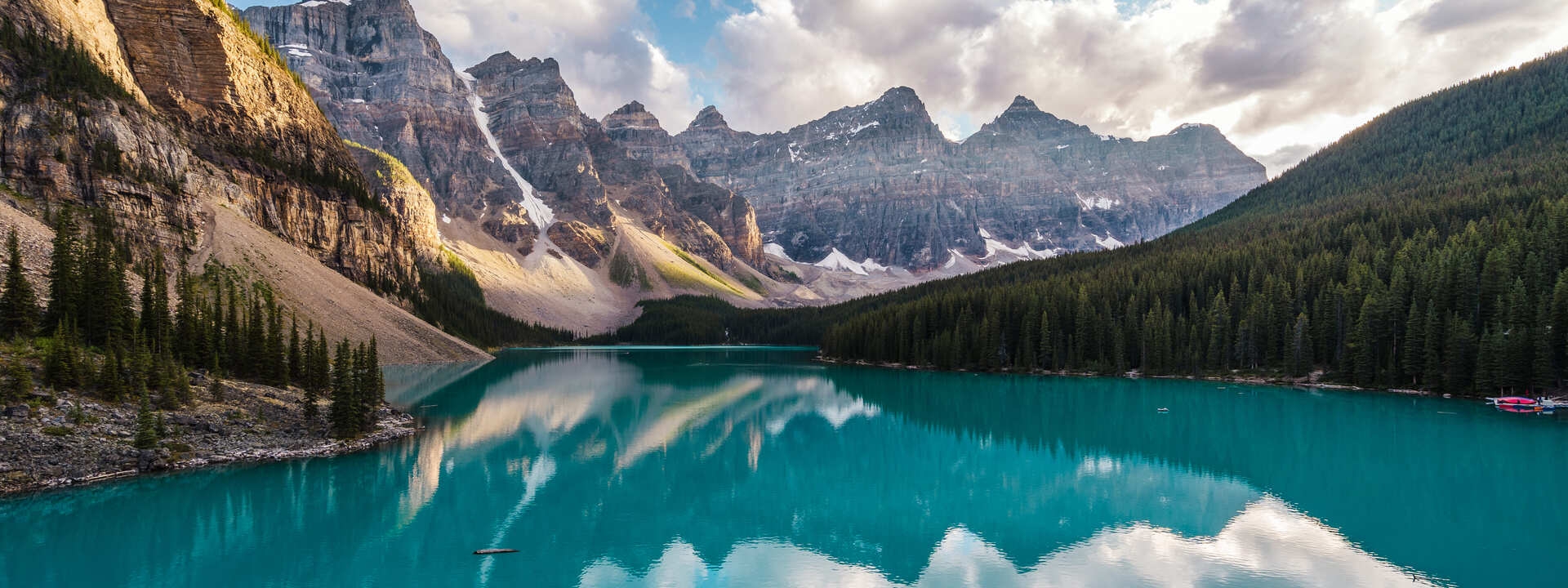This breathtaking landscape image, which could be mistaken for a high-quality photograph or a painting, displays a panoramic view of a serene lake nestled amidst towering, rocky mountains. The large body of water dominates the foreground, its dark teal hue reflecting the encompassing scenery, including the imposing mountains, sporadic trees, and thick, rolling clouds that blanket the sky, with a hint of blue peeking through. To the left, the mountainous terrain is sparsely adorned with trees and dusted with patches of melting snow. In contrast, the right side features dense forests that line the lake's edge. A small red canoe, possibly a kayak, can be spotted near the shoreline on the left, adding a touch of human presence to the otherwise untouched and tranquil scene. The mountains' mirrored reflection on the pristine lake surface enhances the image’s peaceful and almost surreal beauty.